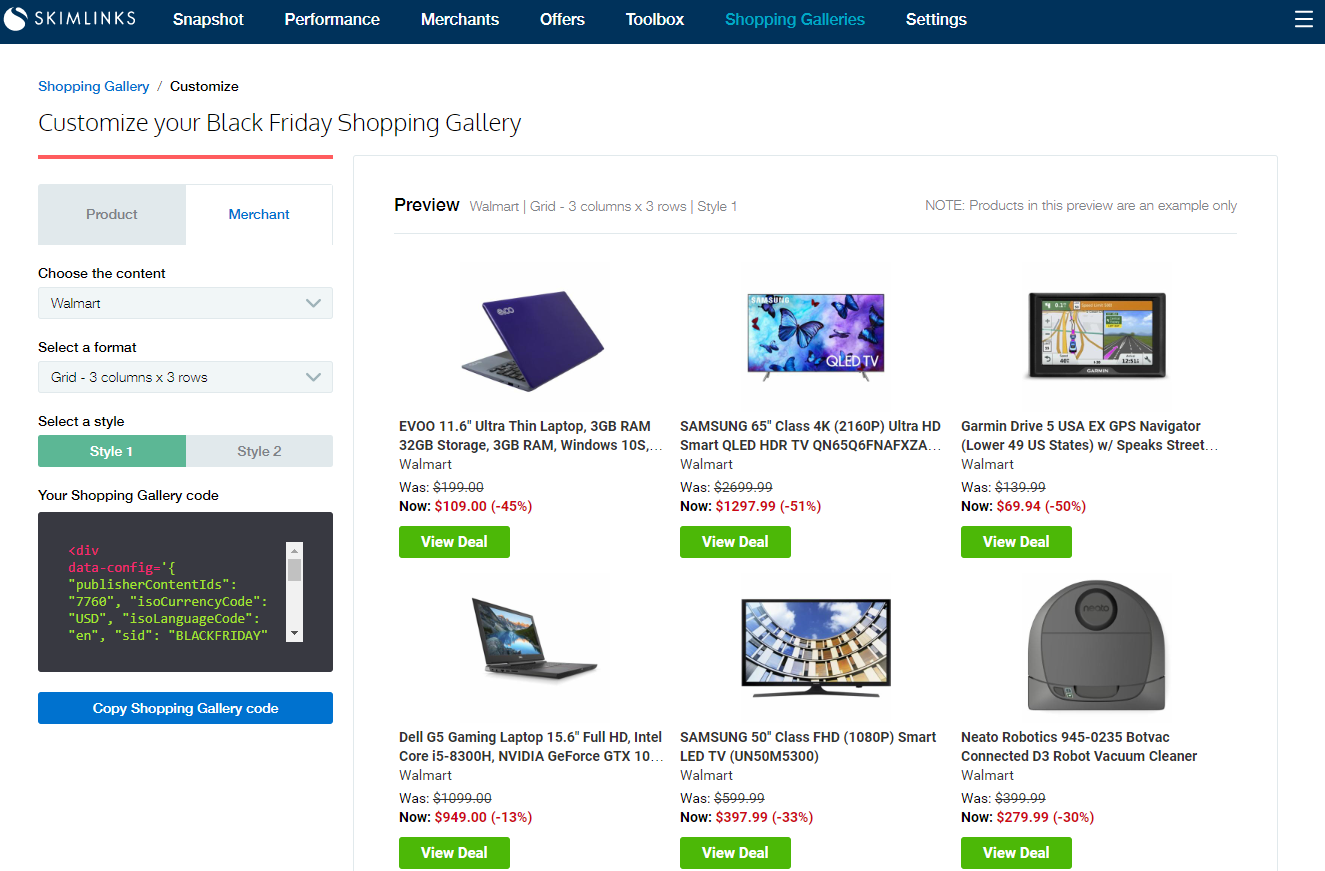The image showcases a Skimlinks website with the "Shopping Galleries" page open, indicated by a blue highlight. 

At the very top, a dark blue navigation bar features the Skimlinks logo on the left, followed by several menu options: Snapshot, Performance, Merchants, Offers, Toolbox, Shopping Galleries, and Settings. On the extreme right, there's a drop-down menu icon. The website's background is predominantly white. 

On the left side, in small blue-highlighted font, it reads "Shopping Gallery / Customize." Beneath this, there's a section labeled "Customize your Black Friday Shopping Gallery," accompanied by a small input window. Here, users can choose between two options: Product and Merchant. This section also includes settings to "Choose the content," "Select the format," "Select the style," and an area for "Your shopping gallery code."

Dominating the right side is a large window labeled "Preview," displaying six products. These products, each with an image, name, and price (original and discounted), are as follows:
1. Evo 11.6 Ultra Thin Laptop
2. Samsung 65-inch Class 4K Ultra HD Smart QLED HDR TV
3. Garmin Drive 5 USA-X GPS Navigator
4. Dell G5 Gaming Laptop
5. Samsung 50-inch TV
6. Neato Robotics Robot Vacuum Cleaner

Each product listing includes a green "View Deal" icon situated beneath the discounted price.